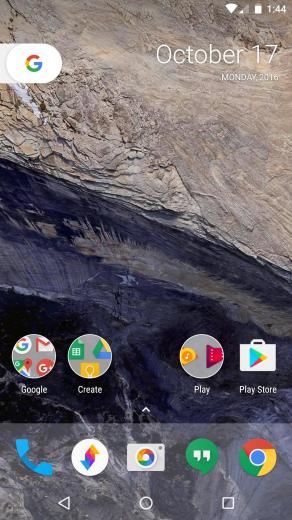The image captures a stunning cliffside scene juxtaposed with a white oval featuring the Google logo in vibrant colors. The date "October 17th, Monday 2016" is prominently displayed, along with the number "144." Various icons are scattered throughout the image: "Google Create," "Play," and "Play Store" are clearly visible. A sleek blue phone is also part of the composition, next to a white circle and a multicolored rectangle. Additionally, icons for a camera, Google Camera, a green chat icon, and the Google Chrome browser are present. At the bottom, navigation symbols including a left arrow, a circle, and a square complete the image.